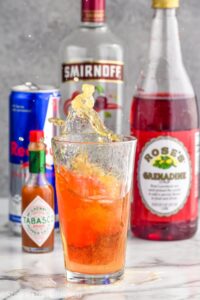In this detailed photograph, a vibrant, orange cocktail is captured mid-splash in a tall, clear glass resembling a rocks glass, situated on a sleek marble countertop. Surrounding the glass are various ingredients presumed to be used in the cocktail's concoction. To the left of the glass is a notable bottle of Tabasco sauce and a blue and silver can of Red Bull. Behind the glass, slightly obscured, stands a bottle of Smirnoff vodka, identifiable by its red cap, though the precise type of vodka is unclear. To the right lies a half-empty bottle of Rose's Grenadine, easily recognized by its red liquid and label. The entire setting, with items placed seemingly at random on the marble surface, hints at a freshly made cocktail with a unique, possibly spicy and energetic blend, perfect for a summer refreshment. A gray background adds a neutral tone to the vibrant scene, ensuring the focus remains on the dynamic splash of the drink and the intriguing mix of ingredients.